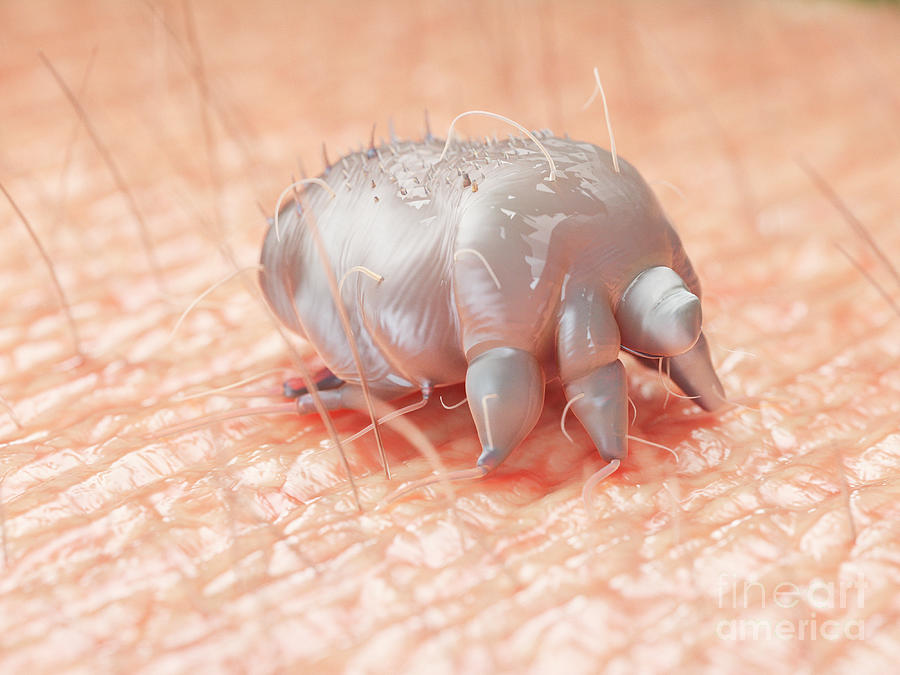The image is an extreme close-up, possibly magnified millions of times, depicting a silver-gray, fleshy mite on human skin. The creature is bloated and appears to be sucking blood, with a red substance visible beneath it on the skin. Its body is slimy and shiny, featuring ruffled lines and prickly protrusions, which might resemble antennae. The mite has three distinct tentacle-like appendages and odd back legs. The skin's texture is rendered in graphic detail, complete with visible pores and hairs emerging from the epidermis, belonging to a person with a light complexion. The overall visual is grotesque, highlighting the mite's unsettlingly detailed appearance against the human skin backdrop.